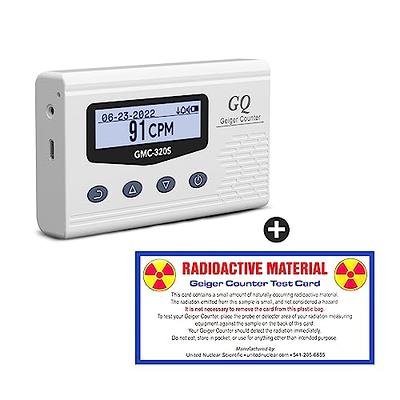This image is a detailed sales ad photo of a GQ GMC-320S Geiger counter, set against a solid white background. The Geiger counter itself is a white, horizontal rectangular device featuring a digital screen with a black border. The screen displays the date "06-23-2022" at the top, the battery life in the upper right corner, and "91 CPM" indicating counts per minute. Below the screen, there are four round buttons: a backup button with a curved arrow, an up button with an upward triangle, a down button with a downward triangle, and a power button. On the right side of the device's face, it reads "GQ Geiger Counter" with the model number "GMC-320S" prominently displayed. The left side of the device houses a USB cord slot, a headphone port, and a sensor hole. 

Additionally, there is a separate blue-bordered card at the bottom of the image, featuring a red and yellow radioactive sign. The card has large, red all-caps text reading "RADIOACTIVE MATERIAL" and below that, "Geiger Counter Test Card" with detailed information in smaller black text.